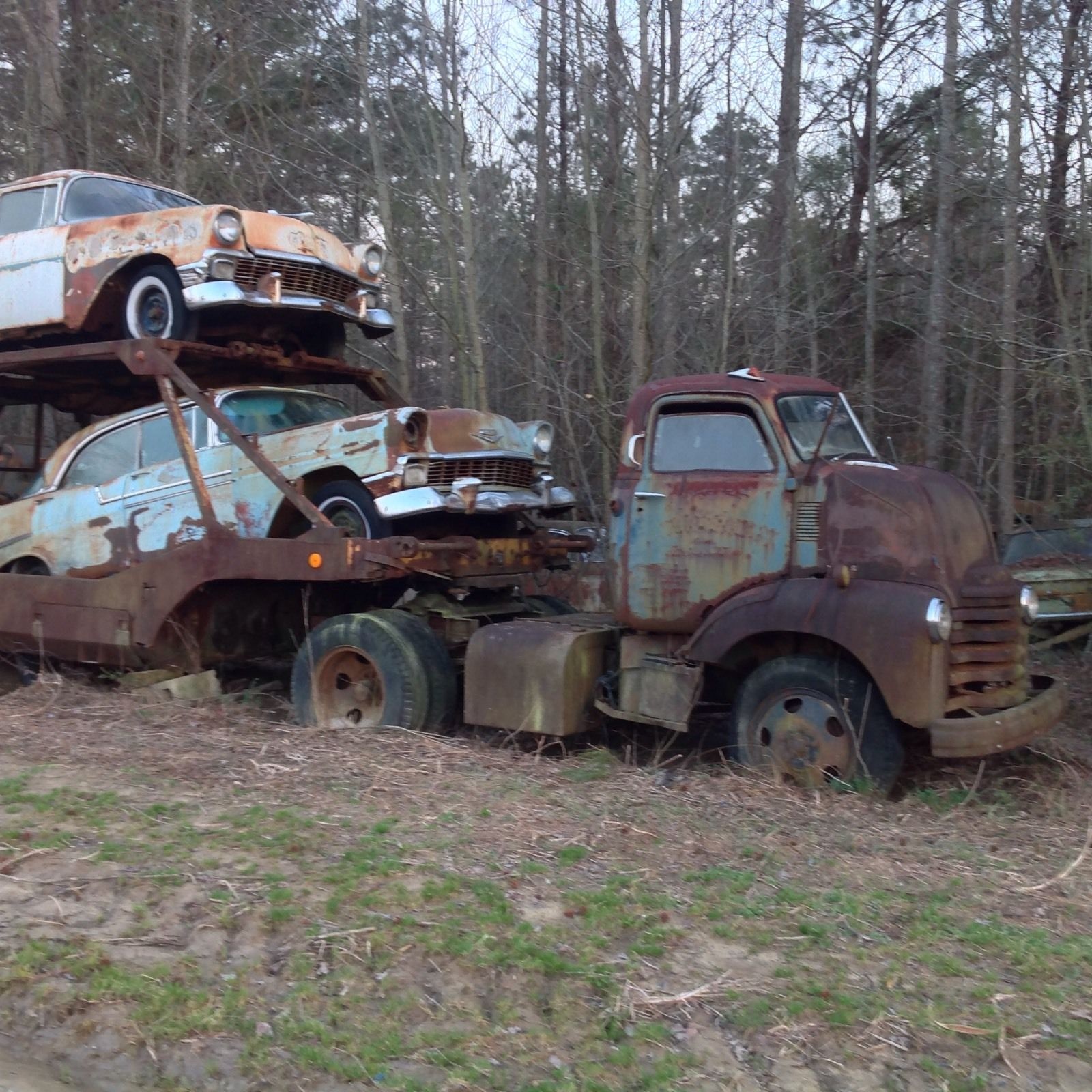This image depicts a heavily rusted and deteriorated tow truck, or car carrier, likely from the 1940s or 1950s, parked in a field near a densely forested area. The truck's cab, with its aqua blue door now succumbing to rust, appears to be sunk slightly into the ground, surrounded by patches of grass and weeds. Attached to the truck is a two-level trailer, equally engulfed in rust, carrying two similarly antiquated and dilapidated cars, one on each level. Both cars, also dating back to the 40s or 50s, mirror the truck’s state of neglect and inactivity, suggesting they have remained stationary for decades. The entire scene exudes an aura of abandonment, with additional worn-out vehicles visible in the periphery, potentially hinting at an old junkyard. The backdrop offers a glimpse of blue sky through the thick canopy of trees, adding to the serene yet melancholic atmosphere of the image.